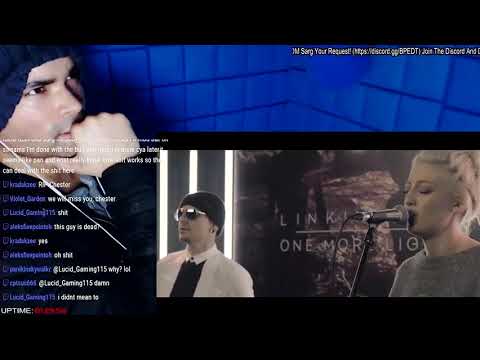This screenshot captures a freeze-frame of a video stream, most likely from a live broadcast as suggested by a persistent chat overlay located on the bottom left of the screen. The chat messages are intermittently appearing and slowly disappearing as they move upwards, indicating active viewer interaction. 

The centerpiece of the image is a man seemingly engrossed in what he is watching. He has his right hand thoughtfully resting on his chin, suggesting a high level of interest or contemplation. Behind him is a blue background, likely soundproofing material, situating him in the corner of a room. He is equipped with a matching blue microphone, adding a hint of professional streaming setup to the scene.

The man is clad in a substantial black jacket and a large hat of either black or blue hue. Wired earbuds run from his ears, further reinforcing the idea that he is deeply engaged with the content.

To his side, on the bottom right corner of the screen, there is a smaller video playing. This video features two individuals performing what appears to be a song: a man on the left and a woman on the right. The partial text "link something morning" suggests the video might be related to a concert or a musical performance, possibly by Linkin Park or a similarly named entity. This implies that the main figure in the screenshot is watching and reacting to this musical performance.